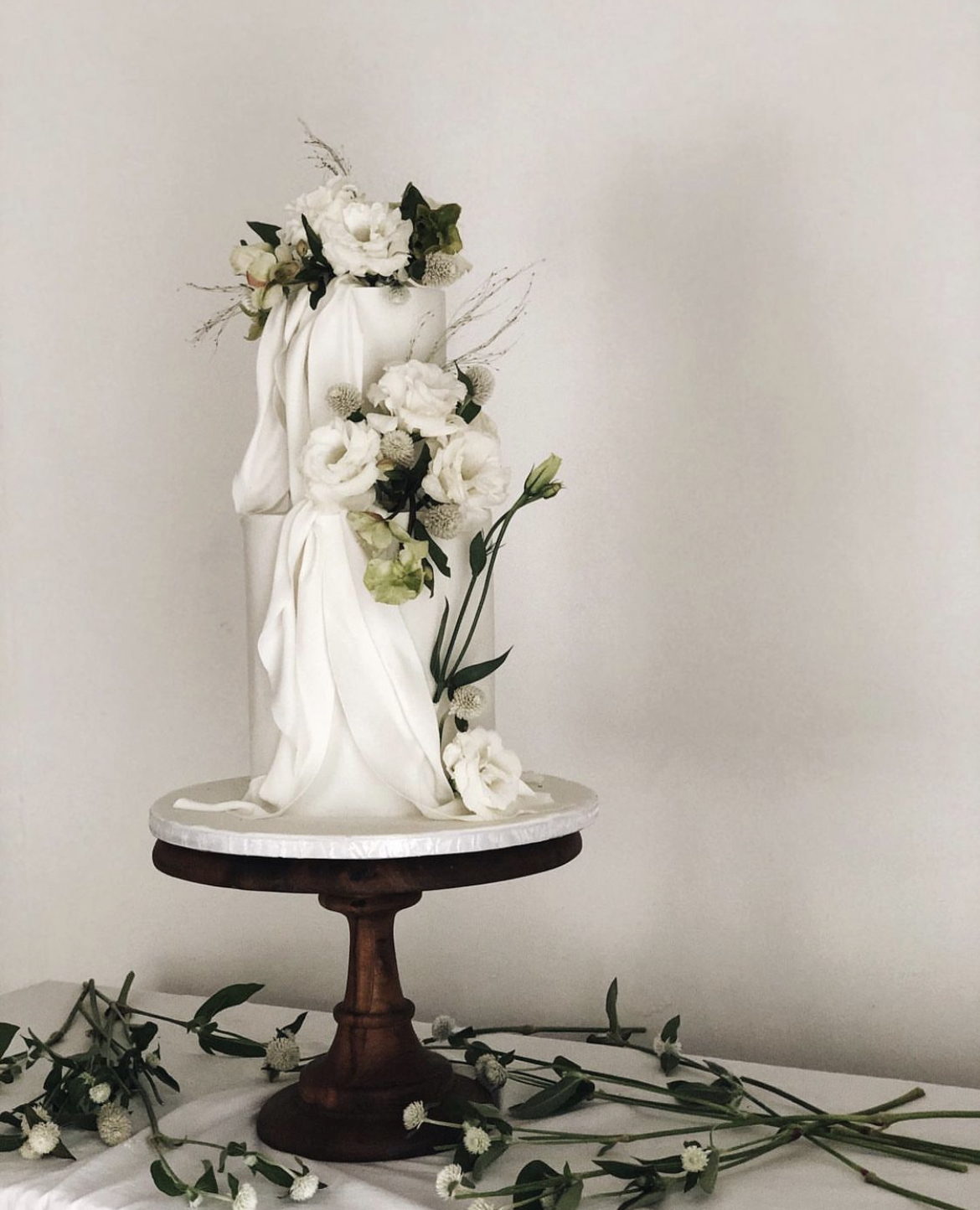This image captures an elegant wedding cake displayed on a sophisticated wooden pedestal cake stand with a white marble top. The cake is adorned with a fondant layer resembling draped fabric, contributing to its delicate and refined appearance. Large white roses, complemented by touches of greenery, embellish the cake, with several roses placed at the top, on the side, and at the base. The stand sits on a table dressed in a white tablecloth, which is further decorated with scattered green stems and small-petaled white flowers. The backdrop is a pure white, casting a soft shadow that enhances the cake's ethereal presentation.